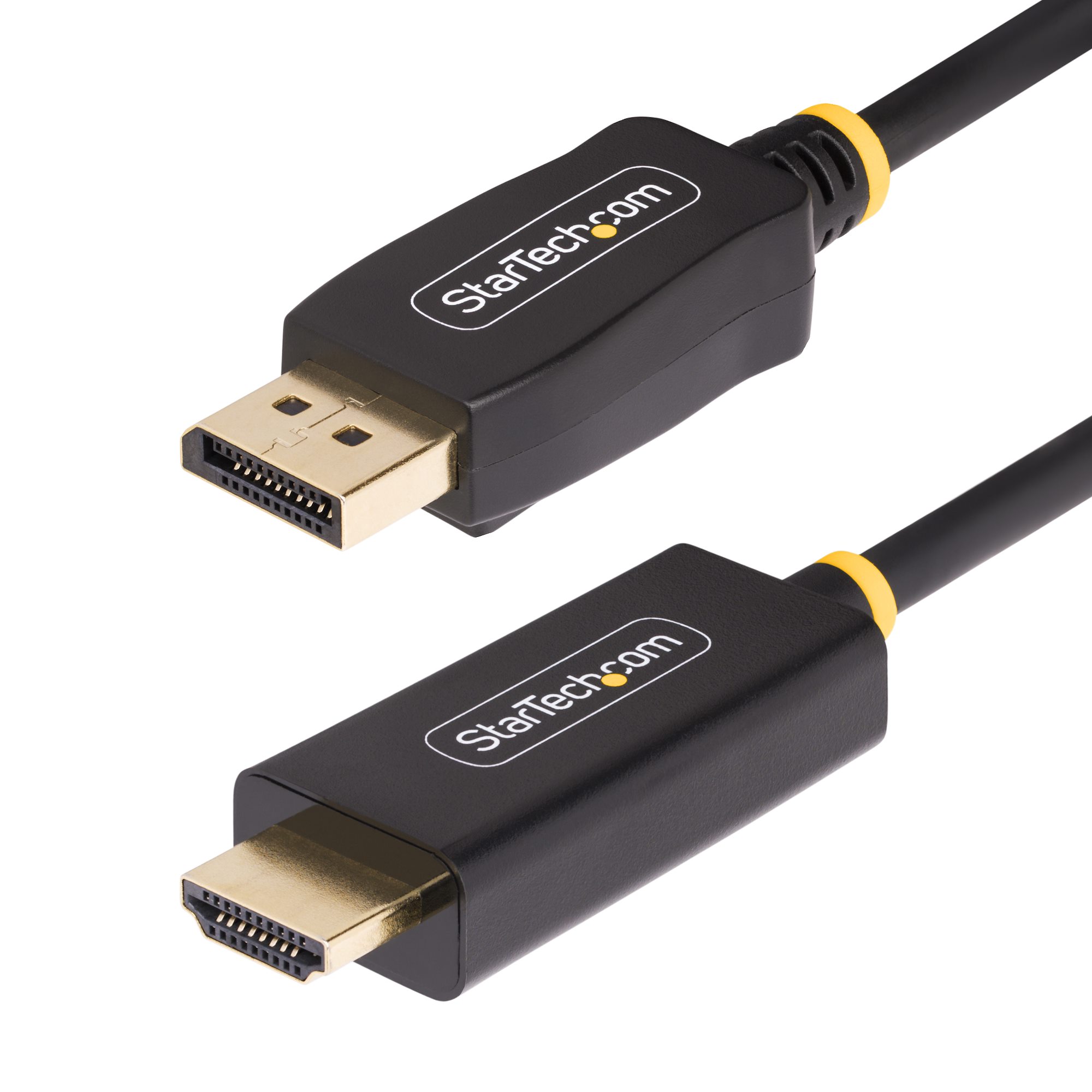This image showcases two diagonally-placed computer cables against a white background. The two cables, identified as a USB cable on the top and an HDMI cable at the bottom, feature connectors encased in black plastic. Both cables display the branding "StarTech.com" in white text, surrounded by an enclosing line, with a distinctive large yellow dot over the ".com" portion. The metallic parts of the connectors are golden in color. The USB cable at the top has a square-shaped connector angled towards the top right corner, while the HDMI cable at the bottom has a sleeker, more rectangular connector angled towards the bottom left corner. The cables extend towards the right side of the image, emphasizing their structured yet slightly varied design.